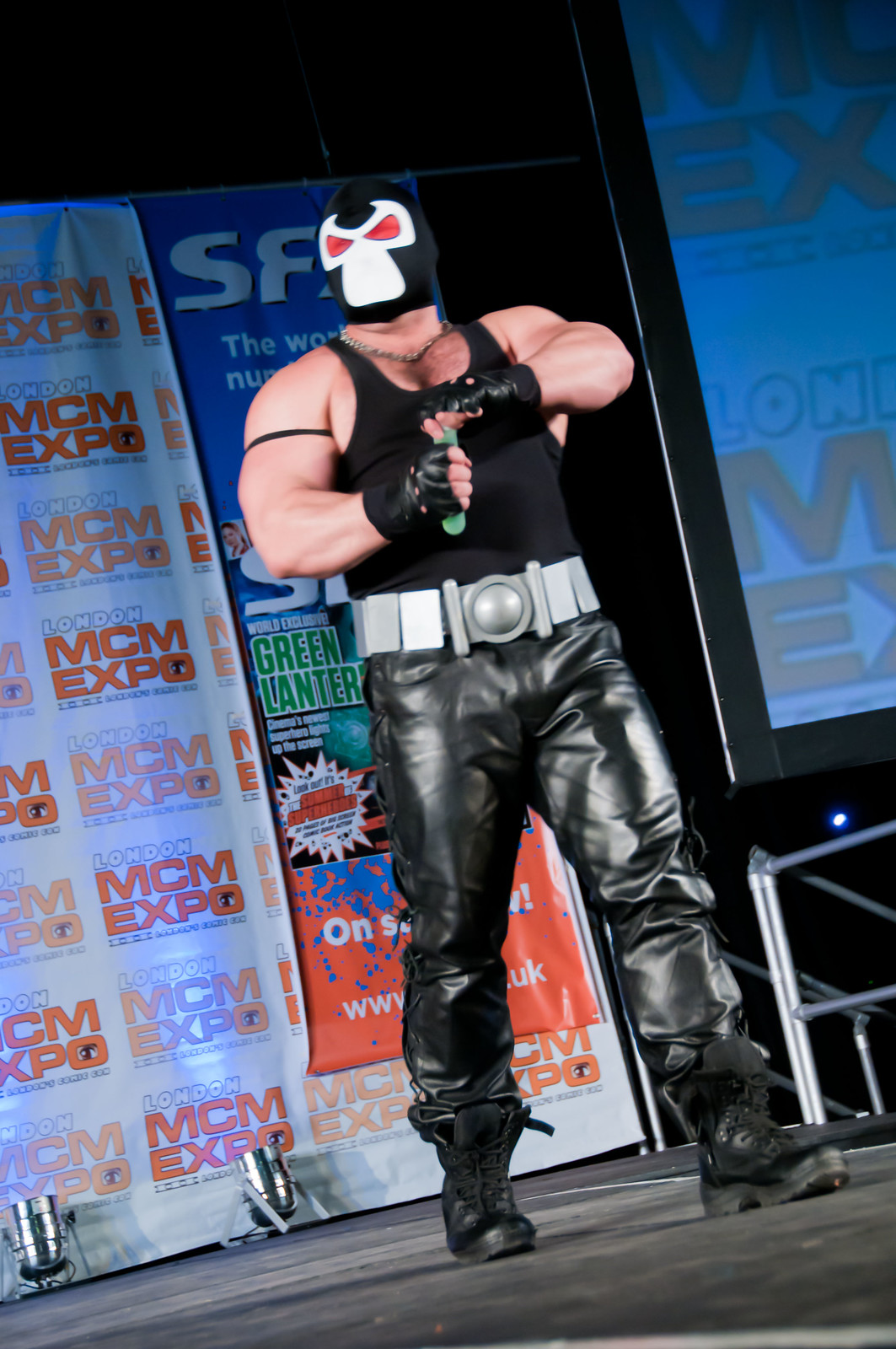This full-color image, though slightly out of focus, captures a muscular individual who appears to be a wrestler, dressed in elaborate fighting attire. The man is wearing black lace-up boots, baggy black leather pants, and a notably thick white or gray belt with a large, prominent buckle. His upper body is clad in a tight black tank top, emphasizing his broad shoulders and muscular arms, one of which features a black band tied around the bicep. His hands are adorned with black fingerless gloves. His face is concealed by a striking mask that closely resembles a skeleton, with a white "quote-unquote" face, red eye holes, and a design that evokes the masks worn by Mexican professional wrestlers, or "luchadores." The wrestler is seen in the act of opening a blue water bottle, suggesting a candid, mid-action capture. He is positioned on a stage, evidenced by a railing in the lower right corner and illuminated by small stage lights on the floor. Behind him, the backdrop features multi-colored signage repeatedly proclaiming "London MCM Expo," establishing both the location and context of the event.